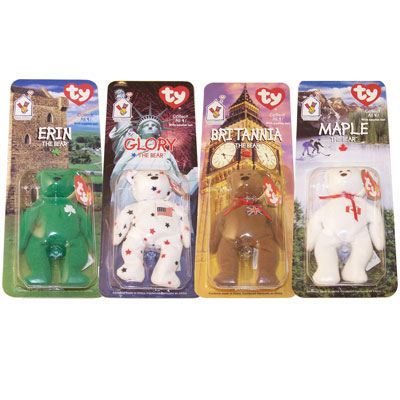This image showcases a collection of four packaged Beanie Babies, each bear designed to represent a different country. The bears are enclosed in clear plastic bubbles attached to distinctive cardboard backings, each adorned with thematic imagery and labeled with the recognizable TY logo—a red heart with white letters—in the upper right corner.

The first bear, named Erin, is green with a white shamrock on its chest. Its package features the Barney Castle in the background. The second bear, Glory, is white with red and blue stars, and it has an American flag on its chest. The background displays the Statue of Liberty and fireworks, emphasizing its U.S. theme. The third bear, Britannia, is brown with a British flag on its chest and a red scarf around its neck. Its backdrop is the iconic Big Ben in London. Lastly, the fourth bear, Maple, is white with a Canadian flag on its chest and a red necktie. The background illustrates a Canadian ice hockey scene, reinforcing its national theme.

Each package prominently displays the name of the bear: Erin in white letters, Glory in red letters, Britannia in white letters, and Maple in white letters, emphasizing their unique identities and national representations.